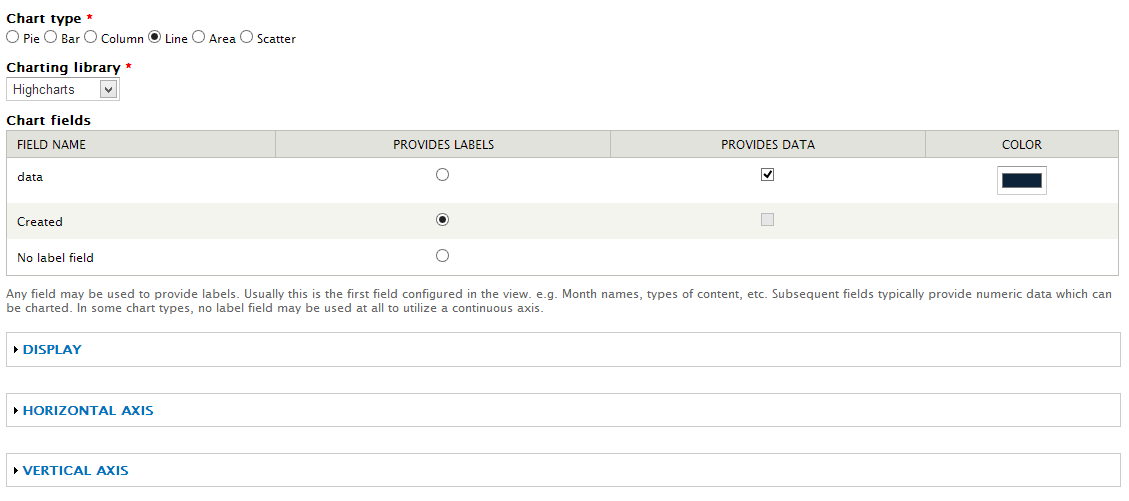This image is a detailed screenshot from a web-based application that enables users to customize data visualizations. The main section allows users to select the chart type from various options including pie, bar, column, line, area, and scatter charts. A drop-down menu is available for choosing the charting library. Additionally, the interface includes a table labeled “Chart Field,” which contains columns for field name, labels, data, and color settings. There are expandable sections for further customization options, specifically for display settings, the horizontal axis, and the vertical axis. The design is minimalist, utilizing mostly black, white, and gray tones. Notably, the screenshot only captures the customization and editing interface, without revealing any actual data or webpage title.